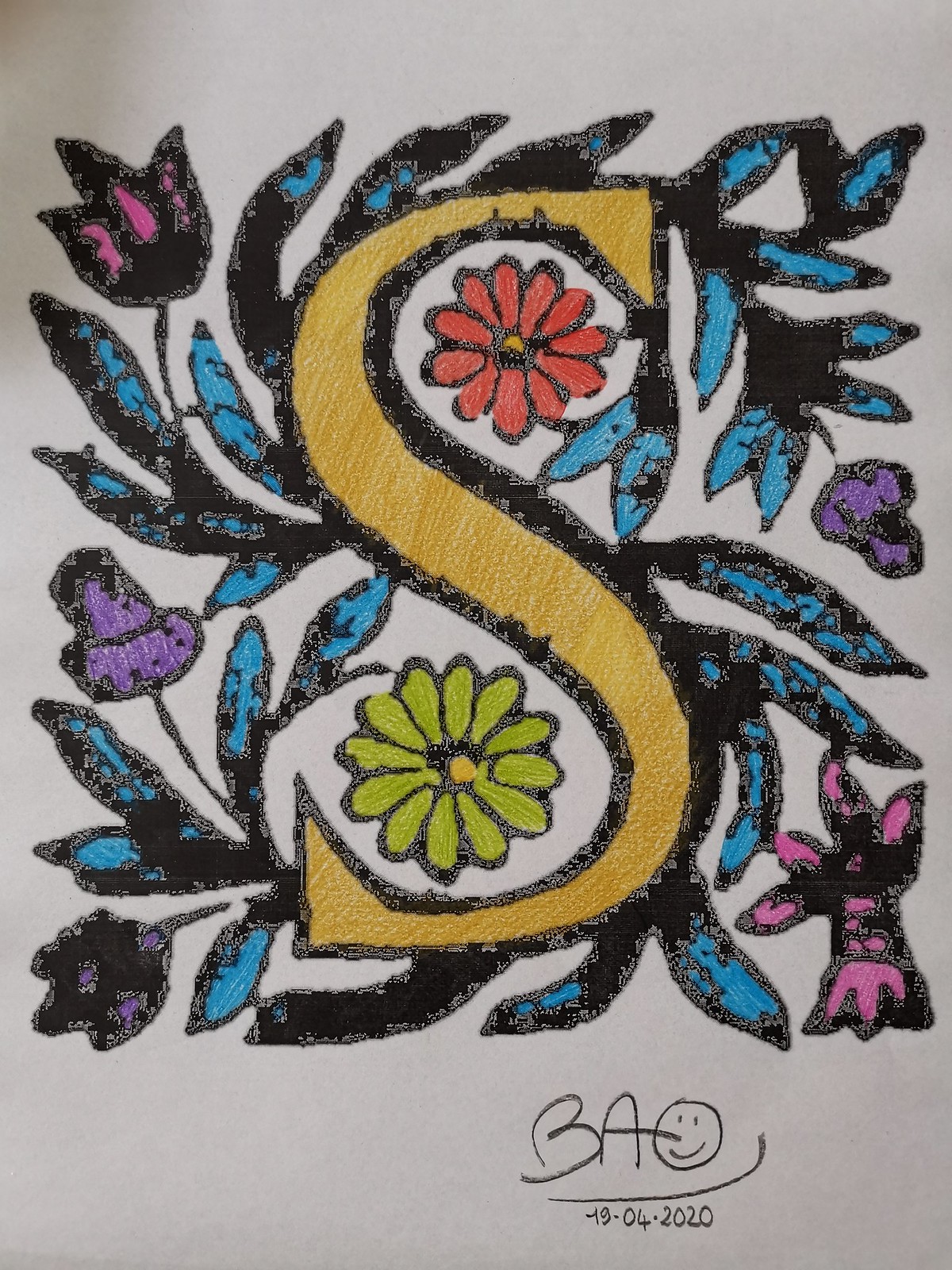This image depicts a vibrant painting centered around a large letter "S" with a dark yellow fill and a black border. The "S" integrates seamlessly with an elaborate botanical theme, featuring intricate floral and leaf designs. Extending from the black-bordered "S" are blue and black leaves, interspersed with various flowers. In the upper curve of the "S" rests a bright red daisy-like flower, while the lower curve showcases a green flower with similar daisy characteristics. Additional flowers, including pink tulip-like blooms and purple flowers, are interwoven among the leaves, suggesting an organic, nature-inspired motif. The painting sits on a white background, enhancing its colorful elements. At the bottom, the artist has signed the piece with "B.A." adorned with a smiley face, and the date, April 19, 2020, indicating its completion.